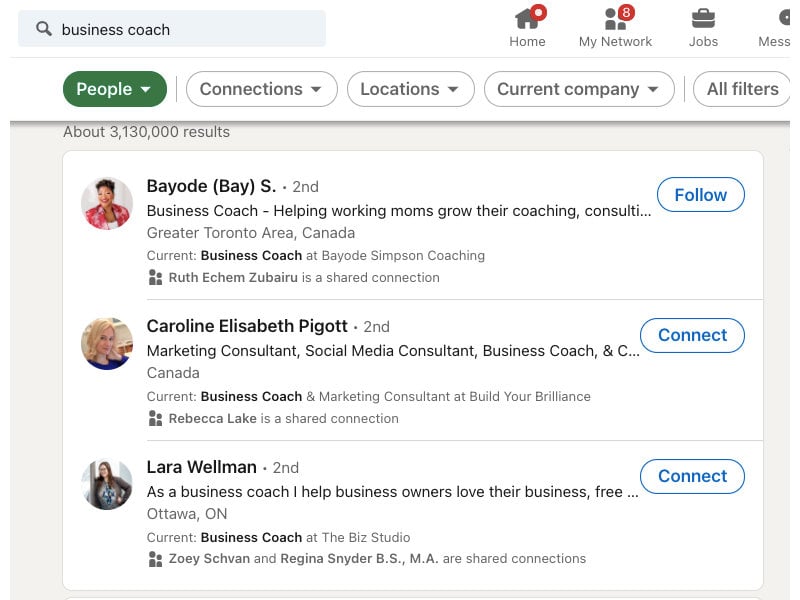Screenshot of a business website featuring a search query for "business coach." At the top left, there is a search bar displaying the entered query. The search yields approximately 3,130,000 results, with the first three visible on the screen.

1. The top result is for "Bayody" (commonly referred to as "Bay"), listed as a business coach specializing in helping working mothers grow their coaching and consultation businesses. The description is partially cut off but indicates Bay is located in the Greater Toronto Area, Canada. Bay currently works at "Bayody Simpson Coaching" and shares a connection with Ruth Eshem Zubaru, a person known to the screenshot taker.

2. The second result features Caroline Elizabeth Pigott, who is identified as a marketing consultant, social media consultant, and business coach.

3. The third result lists Laura Willman as a business coach who assists business owners.

The screenshot provides a snapshot of search results focused on finding a business coach, with a mix of detailed roles and professional connections.